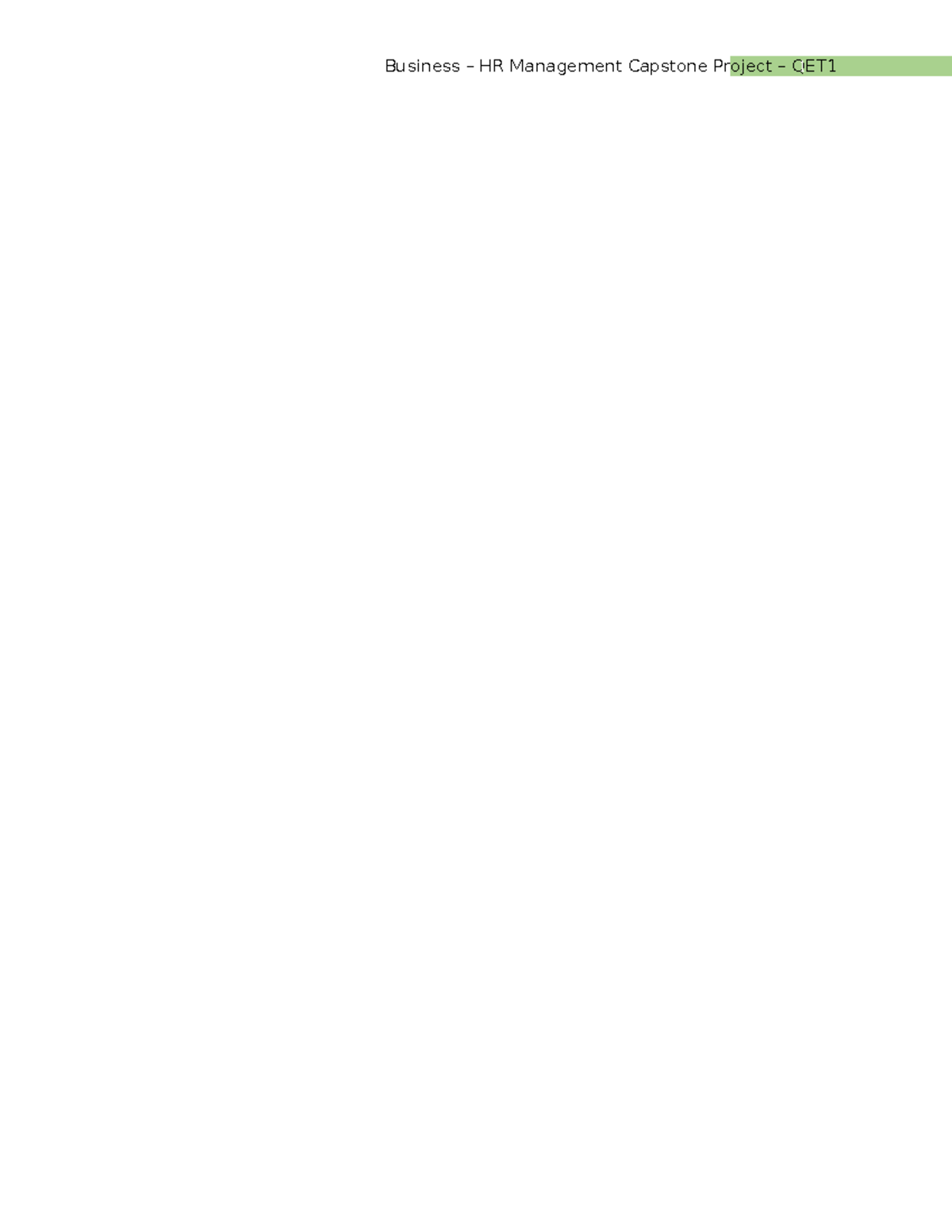A digital screen displays a perplexing document titled "Business/HR Management Capstone Project - QE T1". The title is presented prominently, with each section clearly delineated for emphasis. The text "Project" is highlighted in green, extending slightly beyond its own word boundaries, underlining its importance. The "QE T1" segment appears in capital letters with dashes and spaces separating the elements, enhancing the layout's organized appearance. Despite the well-defined title, no additional content is visible on the screen; the page remains otherwise blank, devoid of further information or context.